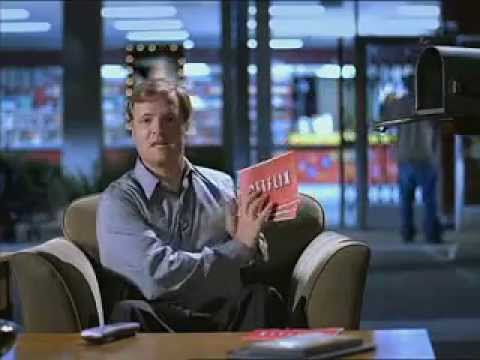In this indoor photograph, a gentleman is seated centrally on a one-seater, light brown or tannish-looking, leather sofa. He is wearing a blue shirt and is looking directly at the camera. The man is holding up three reddish Netflix mailers with white print, showcasing them to the viewers. In front of him is a brown table, on which a remote control and another disc-like item are placed. To his right, there is a dark gray, open letterbox. The background is somewhat blurred but reveals a shop or mall with glass doors and windows. Through the glass, another person wearing a gray jacket and blue jeans can be seen standing, adding depth to the scene. This image feels reminiscent of early Netflix commercial advertisements, capturing a moment of nostalgia for the mail-in DVD service.